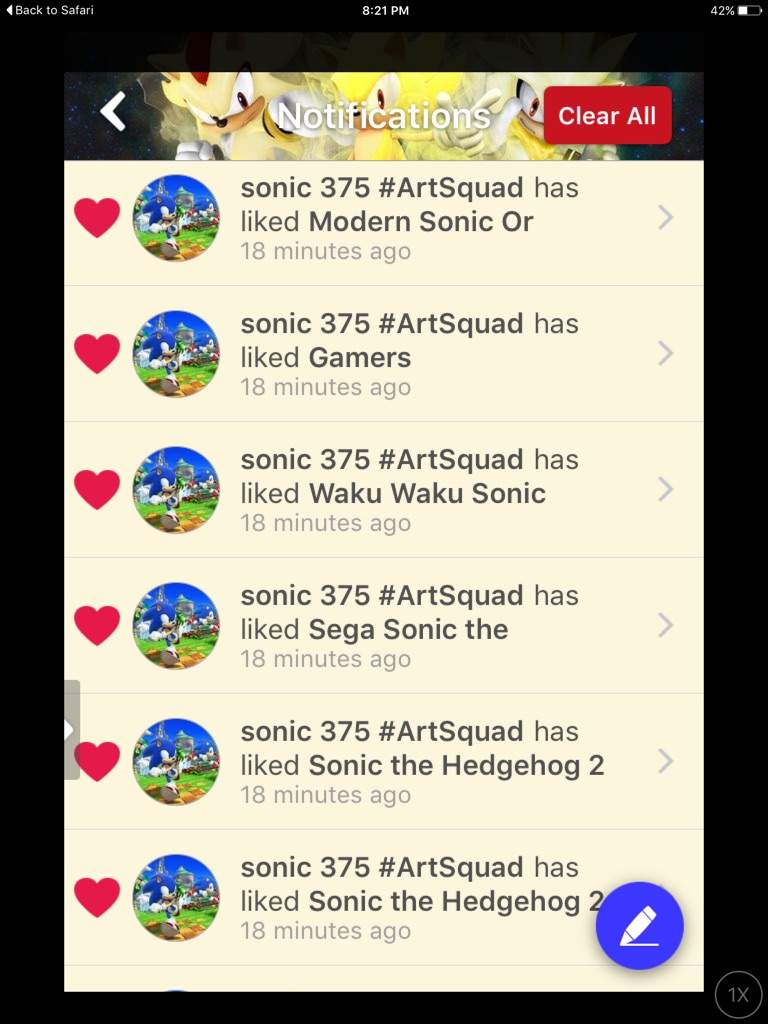The image features a black background with various elements overlaid. In the top left corner, there is the text "Back to Safari," indicating a navigation option. The top middle displays the time "8:21 PM," while the top right corner shows a battery percentage, which appears to be "29%". Directly below this, the word "Notifications" is prominently displayed. The background behind the notifications appears to contain an image resembling Sonic the Hedgehog, but with yellow and tan coloring instead of the iconic blue.

Beneath the notifications heading, there is a red button labeled "Clear All." Below this button, a white box extends across the screen. On the far left side of the white box, there is a column featuring six heart icons. To the right of these hearts are six thumbnail images, which seem to be screenshots of Sonic the Hedgehog.

To the right of the thumbnails, aligned vertically, the text reads as follows:
1. "Sonic 375, Art Squad has modern Sonic or 18 minutes ago"
2. "Sonic 375, Art Squad is like Gamers 18 minutes ago"
3. "Sonic 375, Art Squad is like Waku Waku Sonic"
4. "Sonic 375, Art Squad is like Sega Sonic, duh, 18 minutes ago"

Each line indicates some form of interaction or comment involving Sonic 375 and the Art Squad, with timestamps showing these activities occurred "18 minutes ago."